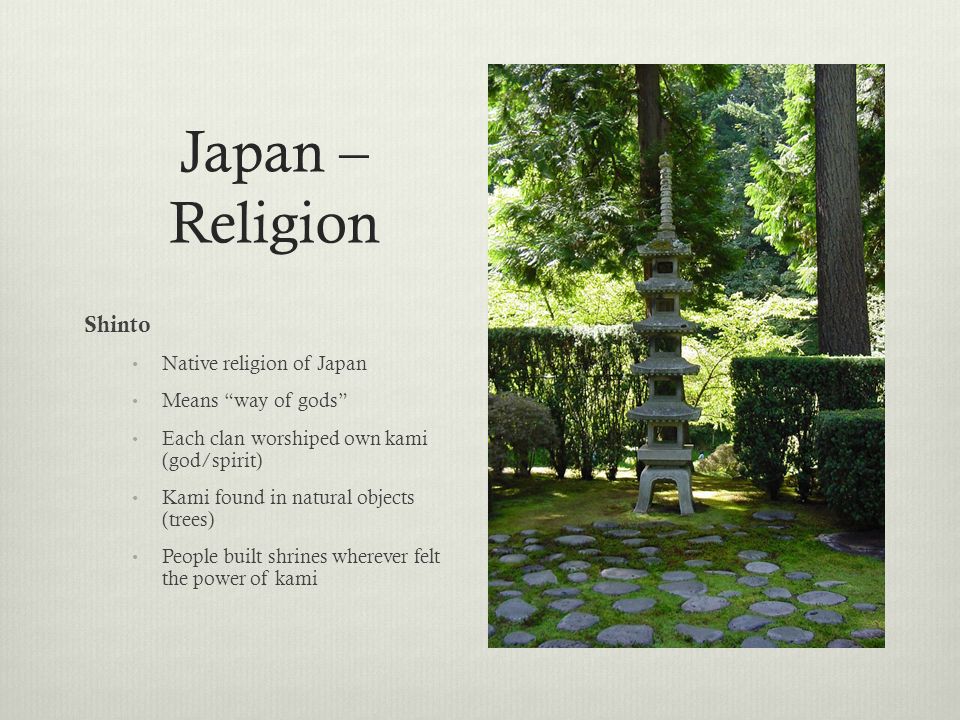The image is a detailed poster depicting a serene Japanese garden. On the left side of the image, the title is prominently displayed: "Japan - Religion," followed by the heading "Shinto" and a series of five bullet points that describe key aspects of Shintoism. The bullet points read: "Native religion of Japan," "Means 'way of gods'," "Each clan worshipped its own kami (god/spirit)," "Kami found in natural objects, such as trees," and "People built shrines whenever they felt the power of kami."

On the right side of the poster is a photograph of a beautifully manicured Japanese garden. The focal point of the garden is a tall, elegant tower composed of five stacked structures, each featuring a triangular comb roof and a square opening. The tower, made of what appears to be a granite-colored material, is surrounded by lush greenery, including several well-trimmed hedges, short bushes, and towering trees in the background. This picturesque setting is further enhanced by paver stones arranged meticulously in front of the tower, contributing to the overall sophisticated and tranquil ambiance reflective of the Shinto tradition.